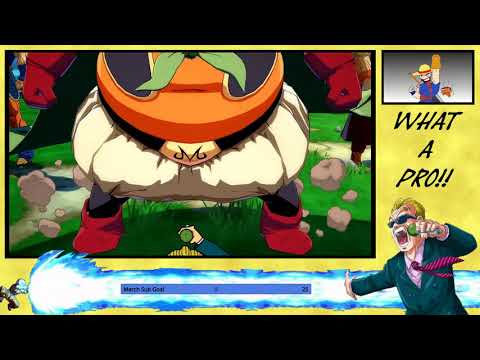The image appears to be a screenshot from a video game with black bars occupying the top and bottom fifths of the screen. The main view is dominated by a close-up of a character's body positioned slightly to the left. This character, standing on a grassy patch, features a chubby physique with a big stomach, wide hips, and thin legs adorned with puffy white pants and red boots. They wear an orange shirt under an ill-fitting blue jacket, a black belt with a gold "M" buckle, and red gloves. You can see a green tie poking out from their belt area. To the right of the main image, there is a smaller rectangular inset, approximately one-fourth the height of the main view. This inset features a character fist-bumping, wearing a blue jacket, brown shirt, and leather gloves, with blonde hair and a bandana. A small creature floats beside him, and the caption below declares "WHAT A PRO!!" in bold caps. Directly beneath this inset, an anime-style announcer with a shocked expression and blonde hair is depicted wearing black sunglasses, a green microphone in his left hand, and a green suit with a red tie blowing in the wind. In the bottom left corner, another character appears to be executing a kamehameha wave maneuver, emitting a large blue blast towards the image's right edge. The overall background is light yellow, and there is some indistinct blue text near the right edge of the image.